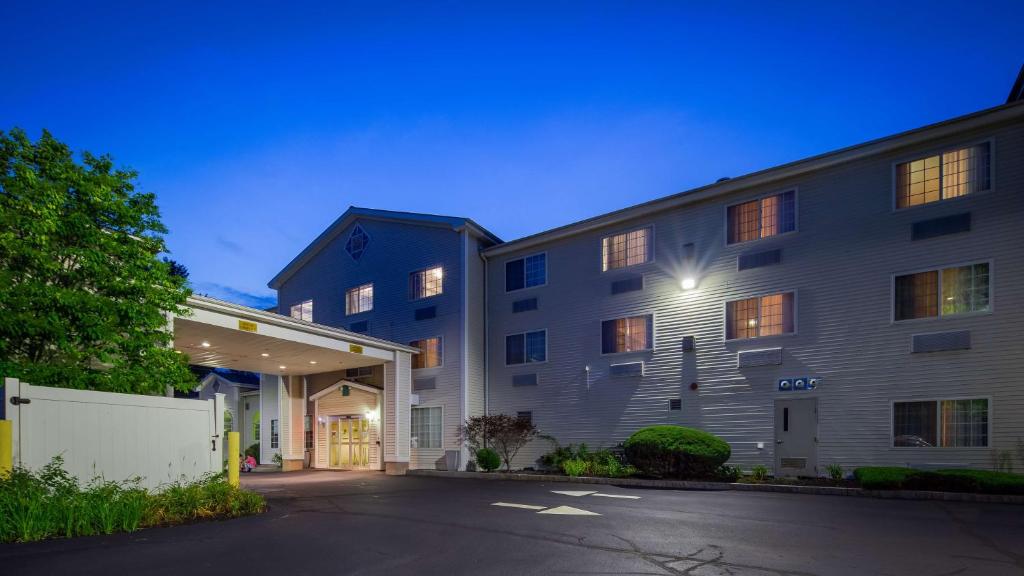The photograph captures an expansive landscape view of a three-story hotel during the transitional period of dawn or dusk, as suggested by the sky transitioning from a dark blue at the top to a lighter hue at the horizon. The foreground features a black pavement parking lot marked with white arrows directing traffic through the hotel's driveway. The building itself, mostly tan in color, dominates the scene with multiple windows, some of which are illuminated, indicating occupied rooms. 

On the left side of the image, an entryway with a canopy extends over the driveway, resembling a typical hotel valet area. This entryway is well-lit with glass doors leading into the lobby. Further to the left, a large green tree is visible behind a white fence, with patches of grass or weeds at its base, adding a touch of greenery to the scene. The hotel's facade is complemented by scattered bushes and noticeable floodlights that illuminate the structure. An emergency exit door is discernible on the right-hand side of the building. The overall ambiance, along with the design and elements, suggests it could be a mid-range hotel similar to a Quality Inn.